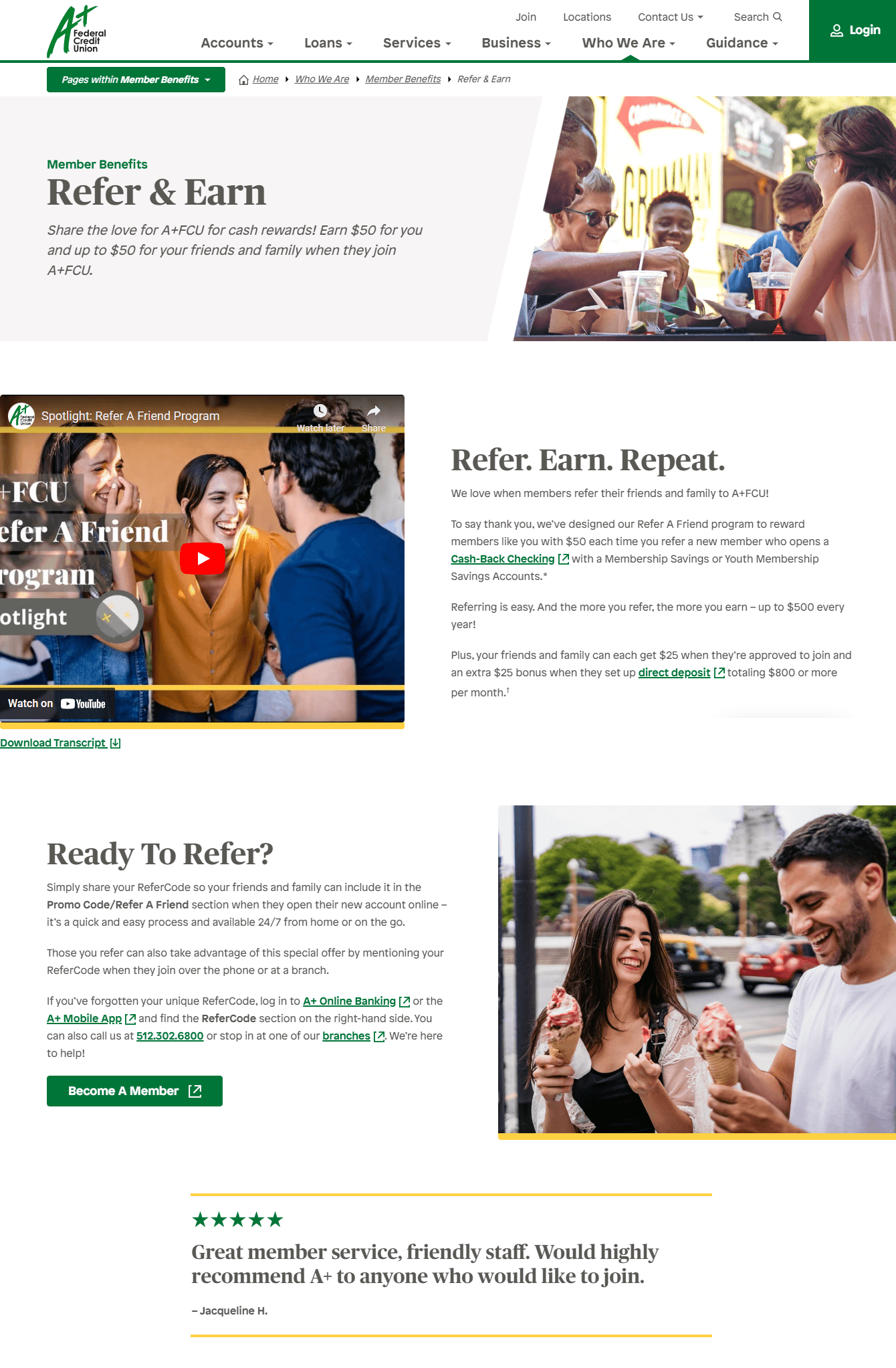Screenshot of the A-Plus Federal Credit Union Website

This screenshot captures the homepage of the A-Plus Federal Credit Union website, showcasing a clean and user-friendly interface characterized by a color scheme of green accents, a white background, and touches of light gray. The typography is predominantly black, ensuring readability against the bright background.

At the top of the webpage, the A-Plus Federal Credit Union logo is prominently displayed on the top left corner. The "A-Plus" text is written in a playful, green, handwritten style reminiscent of a teacher's grade, while "Federal Credit Union" appears in a standard, black font.

The primary navigation menu, located at the top, includes categories: Accounts, Loans, Services, Business, Who We Are, and Guidance. On the far right, a green rectangular button labeled "Login" provides easy access to member accounts. Adjacent to the login button, additional options such as Join, Locations, Contact Us, and Search are available.

Just below the main navigation, a secondary menu is presented in a green box, featuring the phrase "Pages within Member Benefits," along with navigational links to Home, Who We Are, Member Benefits, and Refer and Earn, indicating that the user has navigated to the "Refer and Earn" section.

Central to the screen, within a bordered content area, details about the "Refer and Earn" program are highlighted. On the left side of this section, the text reads:
"Member Benefits
Refer and Earn
Share the love for A-Plus FCU for cash rewards. Earn $50 for you and up to $50 for your friends and family when they join A-Plus FCU."

To the right, a vibrant image features a group of people happily enjoying food and drinks outdoors, enhancing the community feel of the Credit Union.

Beneath this image, a spotlight video about the "Refer a Friend" program is displayed, further explaining the benefits and process. To the right of the video, the text "Refer, Earn, Repeat" introduces the program, accompanied by a brief description and easy access links to related features such as Cash Back Checking and Direct Deposit.

Toward the bottom section, a section titled "Ready to Refer" is presented, which includes additional information on how to become a member, access online banking, and use the mobile app. Essential details about the promo code required for referrals are also provided. Accompanying this text is another cheerful image of two people sharing ice cream, reinforcing the friendly and welcoming ethos of the Credit Union.

At the very bottom of the section, a glowing five-star review from a member named Jacqueline H. adds credibility and positive reinforcement to the referral program.

Overall, the website design is both engaging and informative, effectively communicating the benefits of membership while providing easy navigation and clear call-to-action elements.